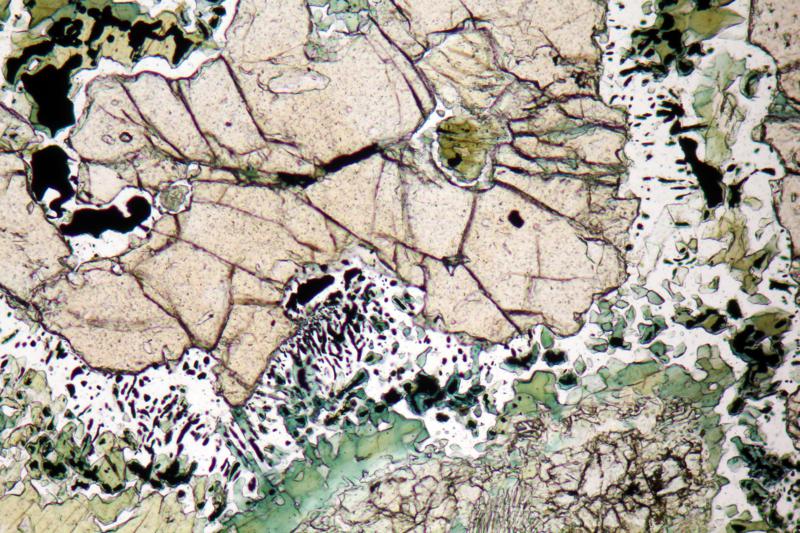This image is a captivating piece of abstract modern art with a marbleized appearance. At first glance, it resembles an aerial photograph of a desert area with an intricate interplay of land and water. The surface is characterized by complex patterns, including white veins with black speckles reminiscent of zebra stripes, distributed across a beige-colored background. Sage green hues infiltrate various portions of the artwork, adding depth and contrast. Towards the lower center, the textures resemble crushed stone, accentuating the piece's rocky appearance. This visually stimulating image invites multiple interpretations, whether it be a detailed microscopic view, an artistic abstraction, or a top-down perspective of the earth's diverse landscapes.